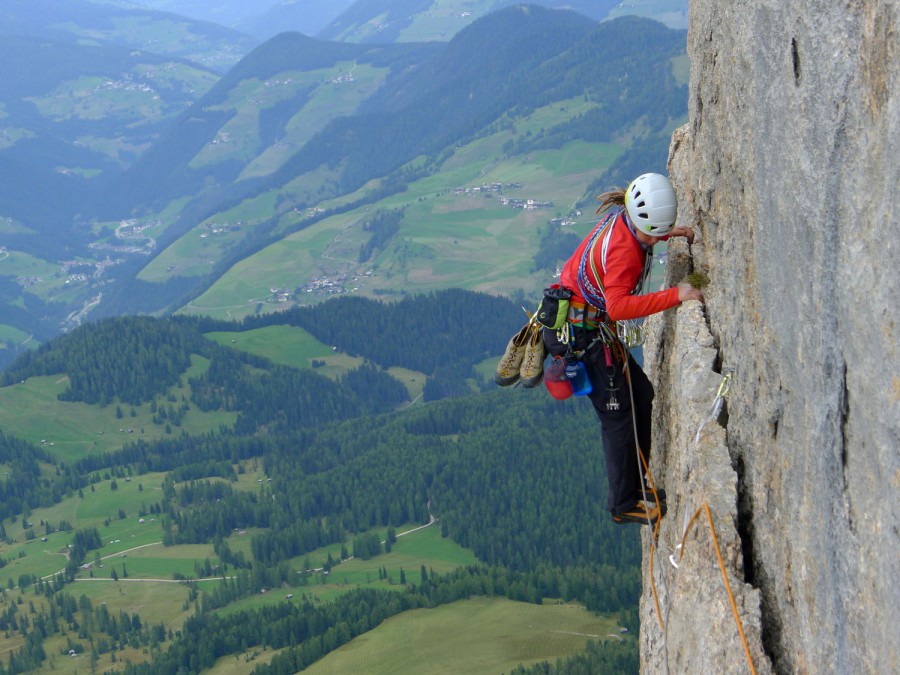This photograph captures a rock climber navigating a sheer granite cliff face, very high above a sprawling valley and mountain range. The climber, positioned on the right side of the image, is dressed in a white helmet with ventilation holes, a red long-sleeved shirt, and black pants. She is seen with her hands wedged into a narrow crack, utilizing technical climbing skills. Her climbing gear includes a utility belt with an extra pair of hiking boots, a blue water bottle, and a bag of climbing chalk. Multiple ropes – orange, gray, and brown – are attached to her side, ensuring her safety. The photo, taken from just above her head, focuses on her ascent and the extensive gear she carries. Below, the landscape reveals green coniferous trees, rolling hills, brown patches of grass, and scattered houses, providing a dramatic backdrop to her adventurous climb.